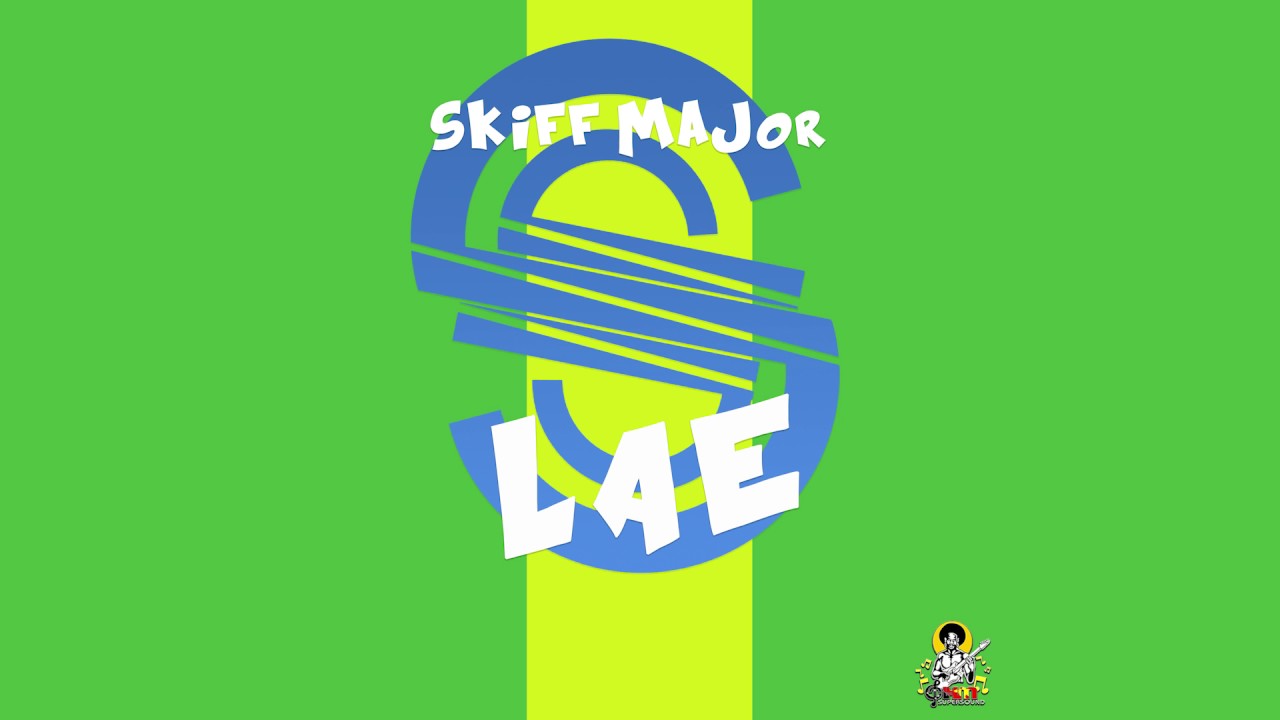The image showcases a logo situated centrally on a background primarily composed of deep green, with a bright lime green vertical stripe running through the center. The main logo, resembling a stylized or playful blue "S" shape, is overlaid with white text that reads "Skiff Major Lay." In the bottom right corner, there's a smaller logo depicting a character, possibly a person or a clown holding a guitar. The color palette includes shades of green, blue, white, black, yellow, and red. The overall composition gives the impression of a flag or brand symbol with a whimsical and vibrant design.